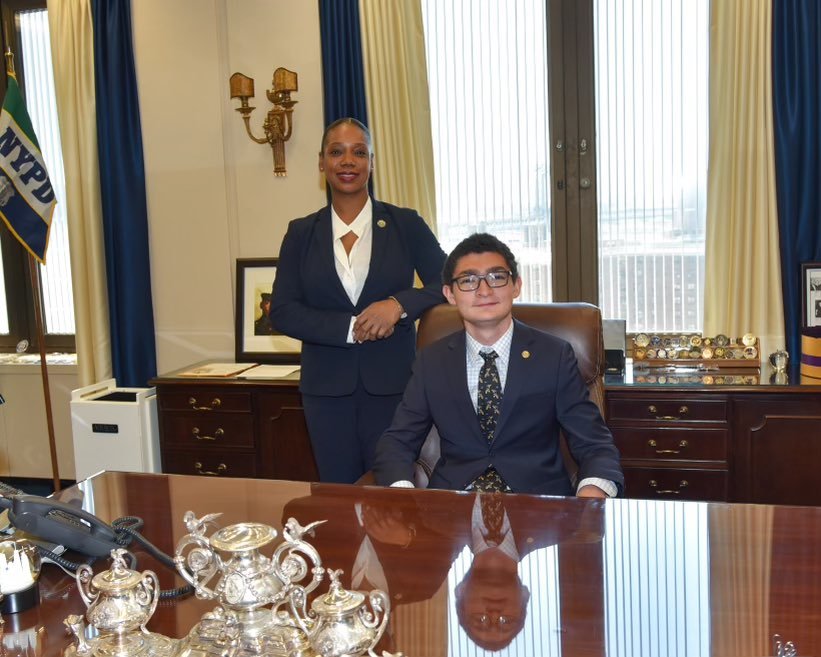The image features an elegantly decorated office setting, highlighting a formal event. At the center, a young Hispanic-looking man, possibly a teenager or in his early twenties, sits at a polished wooden desk in a brown leather chair. He is dressed in a dark blue suit paired with a tie decorated in dark blue and gold floral patterns, a white dress shirt, and a small golden pin on his lapel. He wears glasses and has short dark hair. In front of him, a luxurious silver tea set with ornate etchings and sculptures, including birds, is displayed, indicating luxury and sophistication. A landline phone sits on the desk, and behind him are drawers with a framed photograph and a shelf displaying challenge coins.

Standing behind the young man is an African-American woman, approximately in her 40s, with dark black hair pulled back into a ponytail. She is dressed in a dark blue suit and pants with a white shirt and wears a matching lapel pin. Her left elbow rests on the chair, suggesting a supportive or authoritative presence. A large window adorned with blue and yellow curtains, an old-fashioned antique lamp, and an NYPD flag complete the backdrop. The scene, filled with rich details and personal significance, suggests a setting of professional importance, possibly within a law enforcement or ceremonial context.